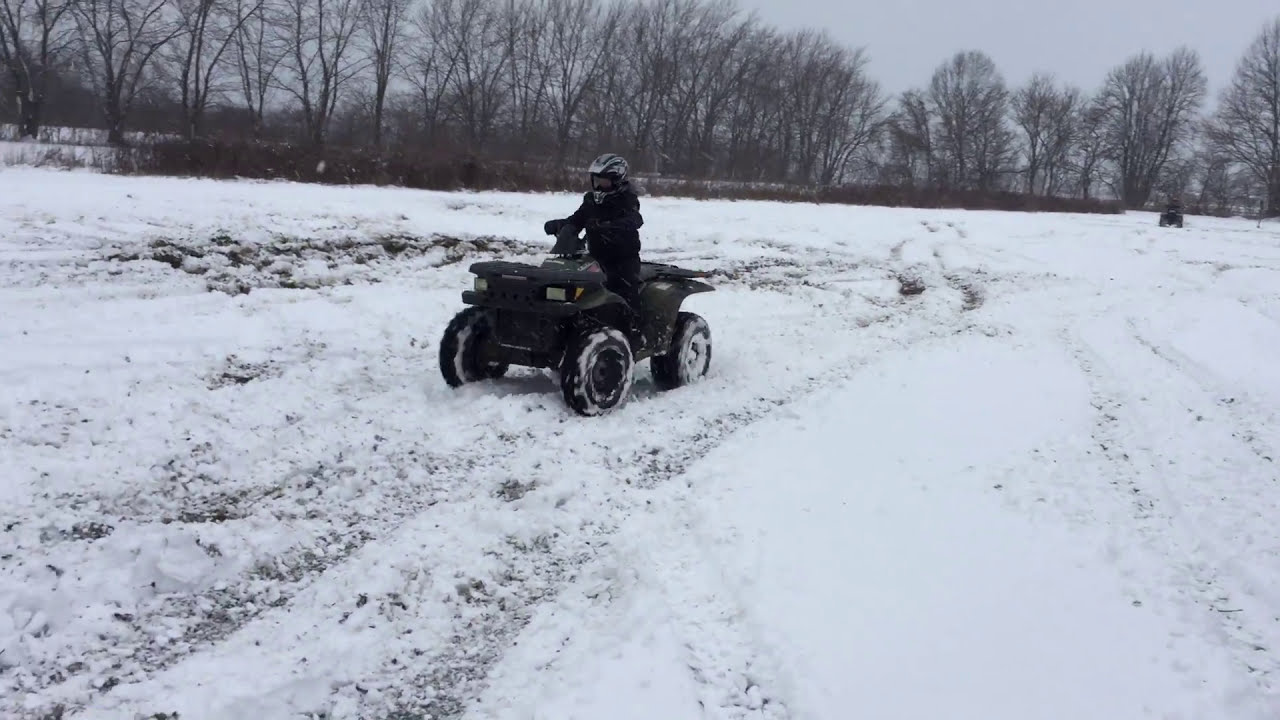In the image, a person clad in dark winter clothing and a full-coverage black-and-white helmet is driving a black four-wheeled ATV through a snow-covered field. The vehicle's tires are caked with snow, and the ATV is traveling towards the lower left-hand corner of the frame, leaving a trail of tracks behind. The snowy landscape reveals patches of dirt and grass. In the background, a tree line of leafless deciduous trees frames the upper part of the scene, accompanied by some brush. The sky is a grayish-blue, devoid of clouds or visible sunlight. Another black ATV can be seen farther back in the image, also marked by tracks in the snow, suggesting previous activity by other vehicles. The serene, wintry environment is void of any buildings or additional people.